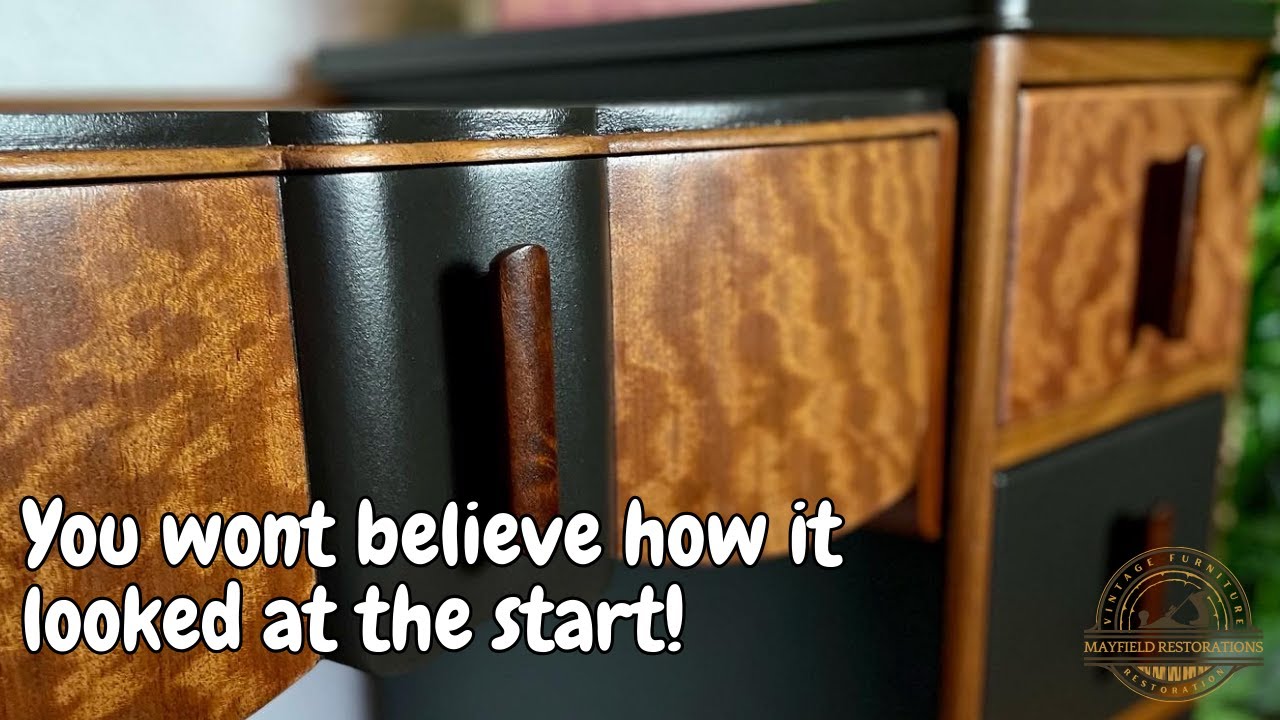This image is a detailed digital photograph of a model train's locomotive, captured in an extreme close-up. The primary colors in the image are dark forest green, black, brown, and light gold. The text "you won't believe how it looked at the start" is prominently displayed in white bubble letters, adding a striking contrast to the scene. The locomotive, though made of plastic, is intricately colored to resemble wood, featuring a brown handle that enhances its realistic appearance. The top part of the locomotive is painted a very dark forest green, while the right side of the image showcases a light gold accent, possibly part of a decorative logo or stamp that is small and somewhat illegible. The bottom of the image features handles, likely designed for donation boxes, adding to the model's detailed craftsmanship. The overall composition highlights the fine details and intricate design of the model, making it a fascinating subject for enthusiasts and casual viewers alike.